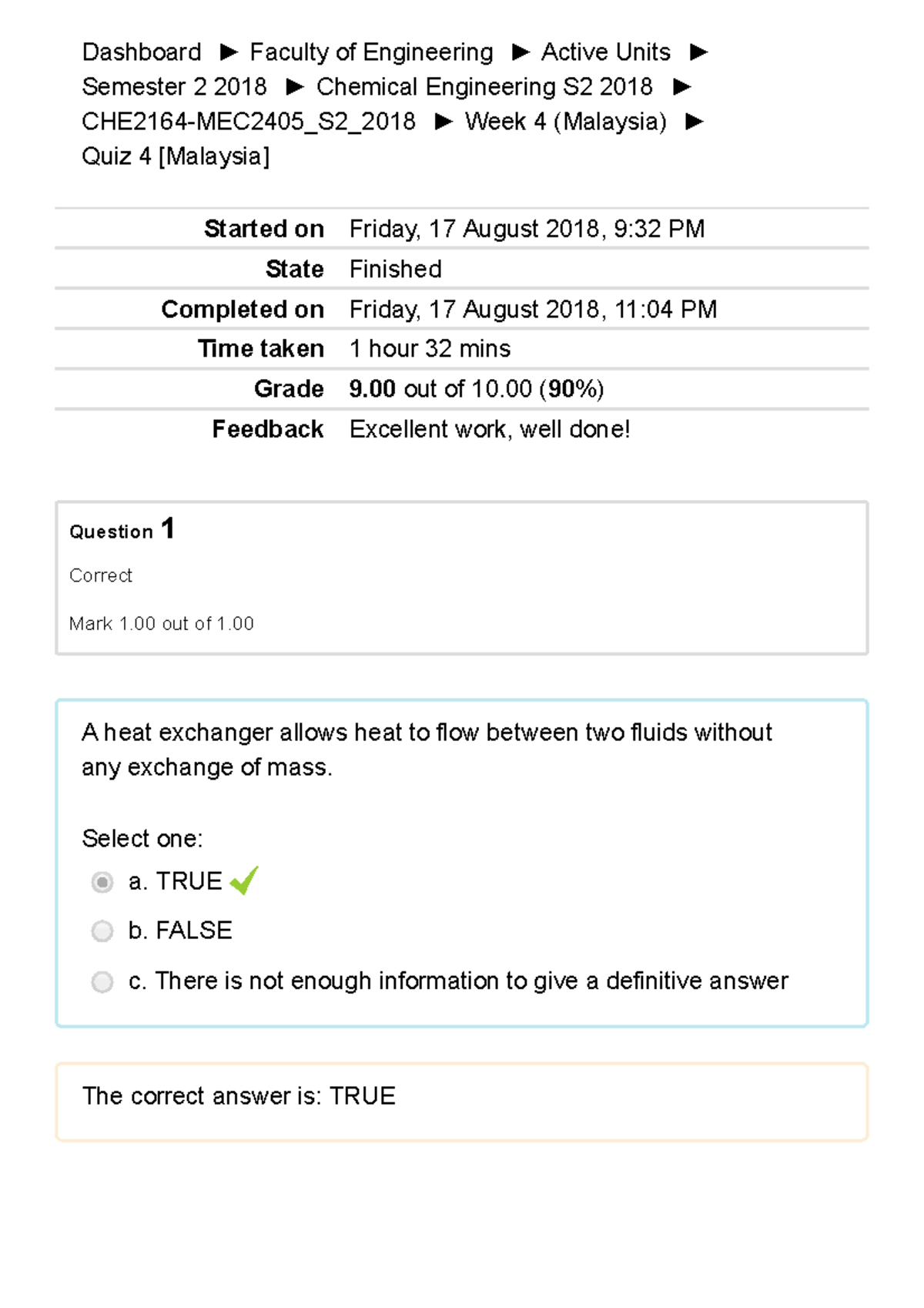This image is a mobile screenshot of a completed quiz interface, likely taken on the user's phone, as suggested by its orientation. The background is entirely white, providing a clear canvas for the black text. At the top of the screen, details of the quiz attempt are presented: 

- **Quiz Start Time:** Friday, 17 August 2018, at 9:32 p.m.
- **Completion Time:** Friday, 17 August 2018, at 11:04 p.m.
- **Duration:** 1 hour and 32 minutes.
- **Grade:** 9.0 out of 10.0, equating to 90%.
- **Feedback:** "Excellent work, well done."

The image focuses on Question One of the quiz, which reads:
"A heat exchanger allows heat to flow between two fluids without any exchange of mass. Select one:
  A. True
  B. False
  C. There is not enough information to give a definitive answer."

A green check mark is visibly placed next to option A, "True." Additionally, a note below confirms that the correct answer is "True." Overall, the screenshot effectively captures a moment of academic success.